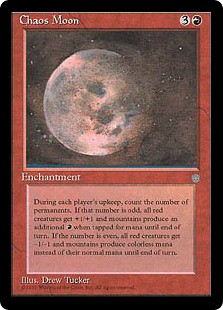This image is a scan of a rectangular trading card, possibly from a game like Magic: The Gathering. The card, titled "Chaos Moon," features a detailed, semi-realistic illustration of a pinkish-gray moon with craters, floating in a starry night sky. Surrounding the moon is a cloud of dust or atmospheric particles, drifting from the right to the left. The card has a thin black border and a deep red background. "Chaos Moon" is written in white text at the top left, with the number "3" and a small symbol at the upper right corner. Below the illustration, the word "Enchantment" is also written in white. The bottom section contains game-related text in black lettering, explaining the card's effect during each player's upkeep: counting the number of permanents and applying specific bonuses to red creatures and mana production. Although the text is blurry and partially obscured, it is clear enough to identify the basic mechanics. The illustration is credited to Drew Tucker, with this acknowledgment appearing at the bottom of the card. The card's overall design suggests it might be an older or well-used edition, adding to its nostalgic and collectible appeal.